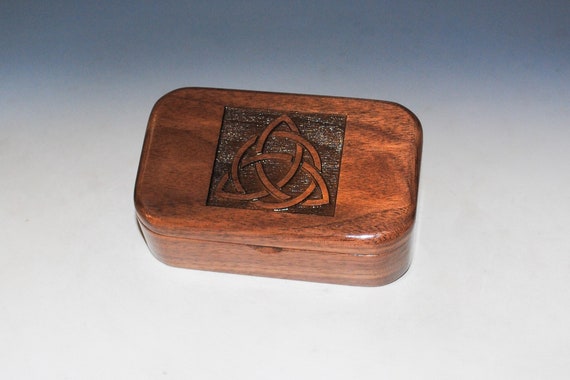The image features a small, wooden box with a smooth, polished finish that gives it a slight sheen. The box is brown and has rounded corners, eschewing the traditional sharp edges. On its top surface, there is a dark square area adorned with a white powdery substance. Within this square, a distinctive symbol is engraved: a circular design comprising interlocking leaf-like shapes. The front of the box includes a small notch, suggesting it could be used to open the box. The background of the image transitions from white at the bottom to a darker blue hue towards the top, providing a subtle gradient that highlights the box’s details.